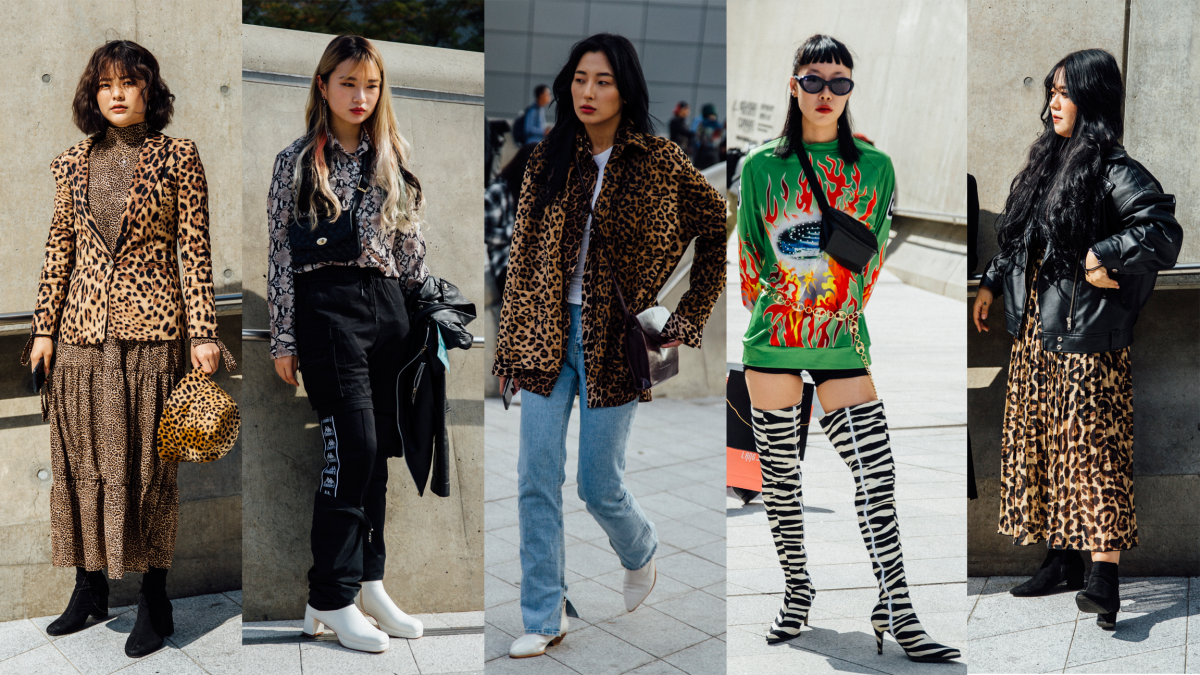The image showcases five young and beautiful Asian fashion models, each styled in various outfits featuring animal prints, standing outside in front of a building. Starting from the left: the first model wears a full leopard print ensemble with a blazer, dress, and bucket hat, complemented by black boots. The second model sports black pants, white boots, a white and black shirt, and has long blondish-brown hair. Positioned centrally, the third model with long black hair is dressed in a leopard print jacket over a white shirt and jeans. The fourth model has medium-length straight black hair, sunglasses, and a green and red shirt, accessorized with a fanny pack around her neck and zebra-striped thigh-high boots. The final model on the right has very long black wavy hair, a black leather jacket, a leopard print skirt, and black boots. The striking combination of different animal prints and fashionable accessories suggests an advertisement or influencer promotion for a vibrant and chic fashion collection.